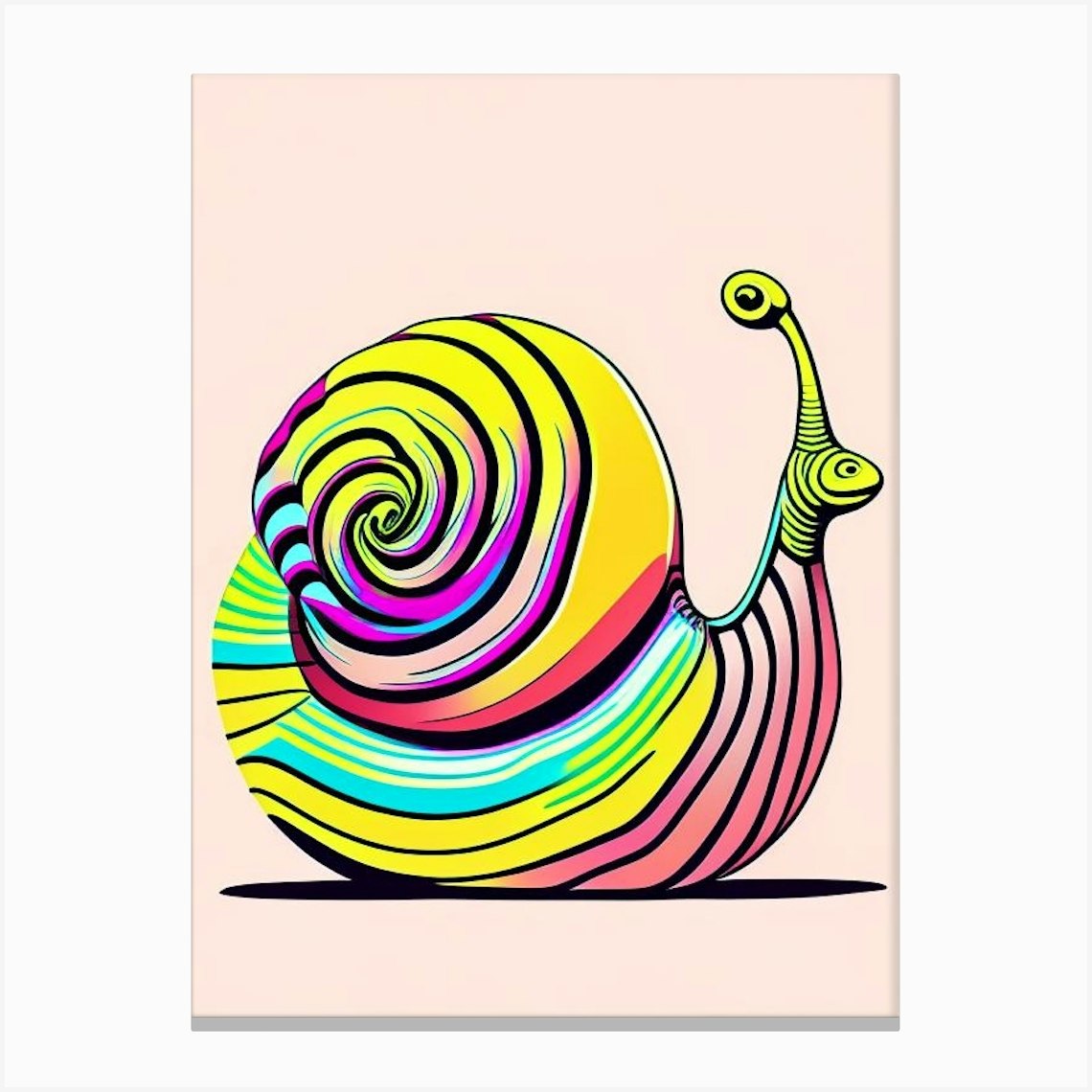The artwork depicts a surrealistic, vibrant snail against a light pink canvas background that resembles the color of salmon. The snail's shell, prominently characterized by its swirling pattern, is primarily bright yellow with hints of magenta, blue, light green, red, and black. The snail's body features an array of vivid colors; its head is yellow with a tooth-like crest at the top, and it has a pink underbelly striped with black. A single antenna with an eye protrudes from its head, and a slight smile can be discerned on its face. The bottom part of its body is pink, giving the impression of the snail scooting without visible legs. Beneath the snail, a dark, circular shadow adds depth to the otherwise fantastical and highly stylized depiction. This highly detailed and imaginative rendition merges elements of realism, such as the snail's signature shell and body, with a striking palette and playful composition, creating an engaging visual experience.